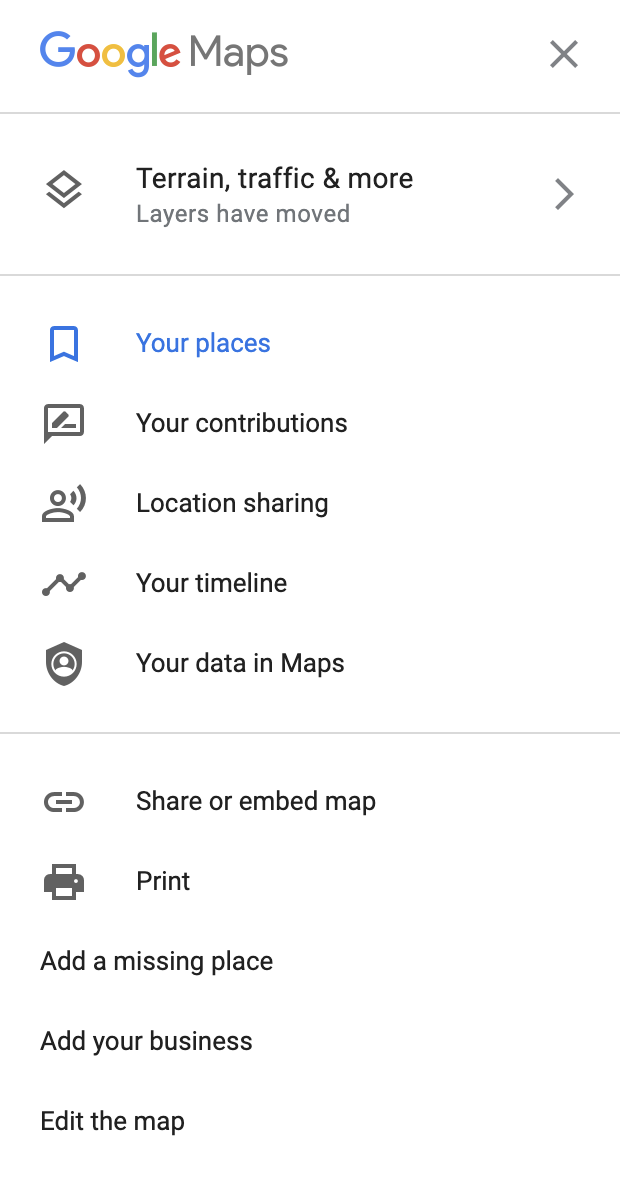This image showcases a section of the Google Maps interface. At the top, the iconic Google logo is displayed, with each letter in the word "Google" colored distinctively: the "G" is blue, the first "o" is red, the second "o" is yellow, the second "G" is blue, the "L" is green, and the "E" is red, while the word "Maps" is in gray. To the right of this, there is an X button. Beneath the Google Maps title, a thin gray line separates the header from the rest of the interface.

Below the line, options like "Terrain," "Traffic," and "More" are visible. There is also a notification that "Layers have moved," accompanied by a bright gray arrow. The section titled "Your Places" is highlighted in blue font, followed by other options in gray: "Your Contributions," "Location Sharing," "Your Timeline," "Your Data in Maps." Another thin gray line separates these options from the subsequent list, which includes "Share or Embed Map," "Print," "Add a Missing Place," "Add Your Business," and "Edit the Map." The background of the entire interface is white, providing a clean and organized look.